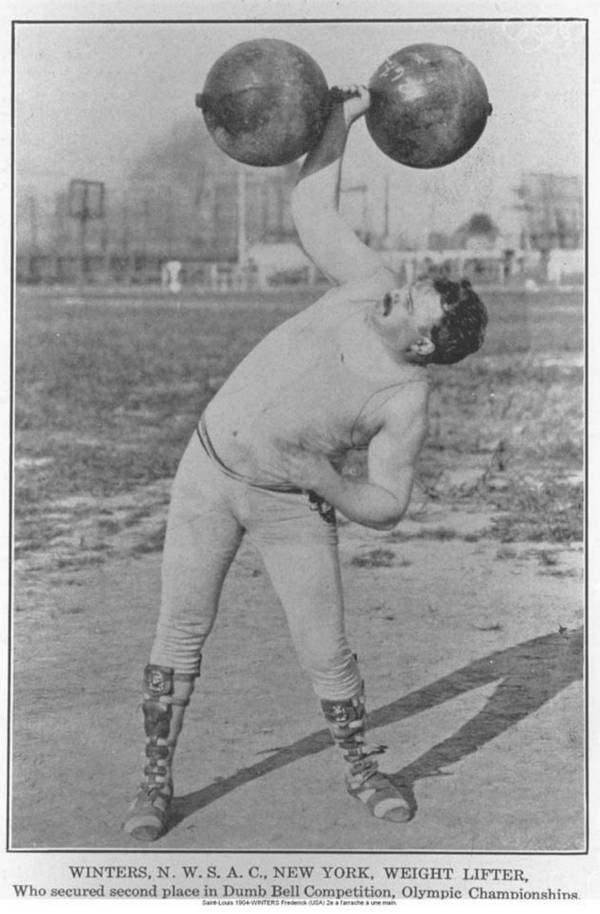This is a faded black and white image of a muscular Caucasian male weightlifter with dark hair and a mustache, standing in a grassy field with a fence in the background. He is centrally positioned in the photograph, wearing a tight tank top, pants, and high-top boots laced up to below his knees. The weightlifter is holding a large barbell with his right hand above his head while his left hand is near his belly. His body is slightly leaned over to the right with his legs spread apart, standing on a dirt patch. At the bottom of the image, there is a caption in black print on a gray background that reads, "Winters NWSAC New York Weightlifter, who secured second place in dumbbell competition Olympic championships." The overall style and tone of the image indicate that it is very old, potentially lifted from a vintage advertisement or magazine, and the scene is clearly sports-oriented.